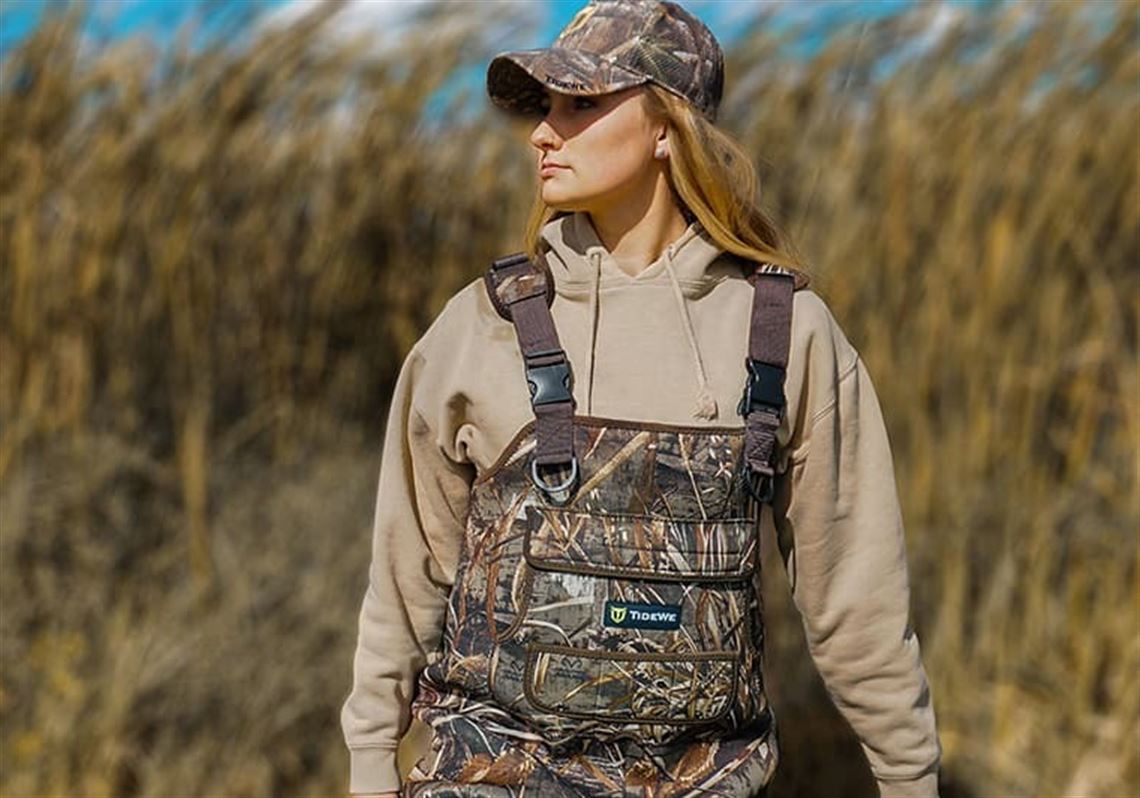This image captures a young Caucasian woman in her mid to late 20s, standing in a field, presumably for hunting given her attire. She is wearing a beige long sleeve hoodie underneath camouflage overalls and a matching camouflage baseball hat. Her long blondish-brown hair flows from beneath the hat, and a shadow from its rim partially obscures her face. The woman is facing forward from the waist up, but her head is turned to the side, offering a profile view of her face adorned with a pearl earring in her left ear. The background, though blurry, reveals a blue sky and what appears to be a field with tall stalks of either wheat or corn, casting a natural, serene atmosphere around her.